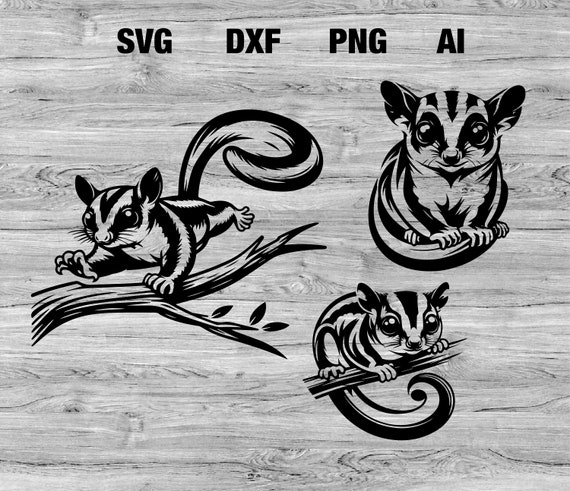This digital advertisement showcases clipart images available in multiple formats, specifically SVG, DXF, PNG, and AI, as indicated by the medium-sized, black, capitalized letters displayed across the top against an ash-colored, whitewashed wood background. The artwork features three black and white illustrated squirrels depicting various positions on the same wood backdrop. The first squirrel on the left is in motion, running across a branch. The second squirrel, centered, is sitting with its tail curled in front, seemingly resting. The third squirrel to the right is hanging onto a branch with its tail dangling below. The highly detailed illustrations are rendered in shades of black, white, and gray, appearing as though they were drawn with a black Sharpie marker.